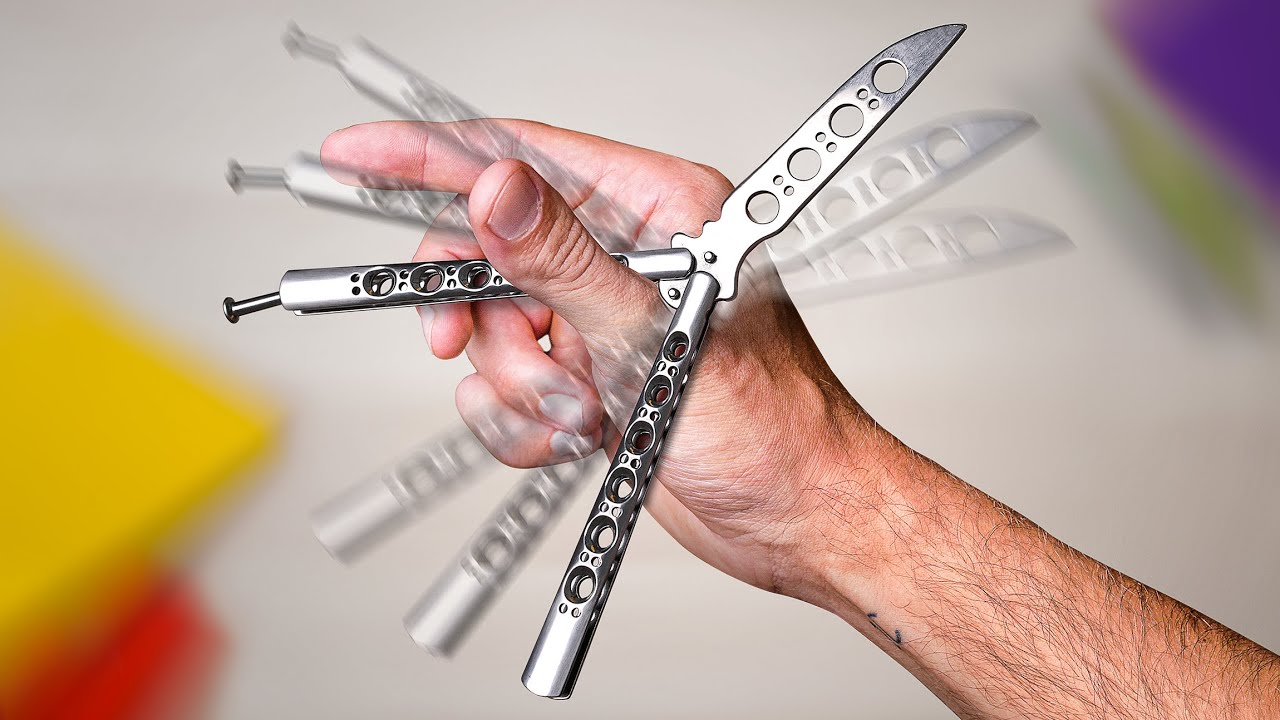In this image, a white man with a hairy forearm is skillfully spinning a butterfly knife. His hand, emerging from the bottom right corner, is positioned with his thumb up and his pointer finger outstretched, while the other fingers are curled back. The intricately designed butterfly knife, which features stainless steel handles each perforated with three holes and two indented dots beneath the larger ones, is grasped between his thumb and forefinger. The blade itself, adorned with four large holes and two indented dots in the middle, extends out perpendicularly to his forearm. A faint tattoo with a letter is visible on the man's wrist. The beige-colored background behind his hand creates a neutral setting, while a purple square shape appears faintly in the top right corner, and yellow and red square shapes are located in the bottom left, all of which are blurry, suggesting the rapid motion of spinning the knife. Multiple semi-transparent, blurry outlines of the butterfly knife emphasize the swift, proficient motion. The image captures the dynamic reflections and shadows cast by the spinning knife, illustrating the motion and efficiency with which it is being twirled.